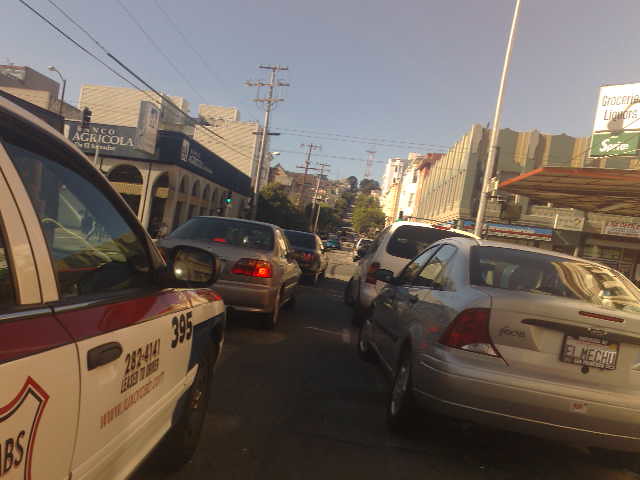The image captures a daytime scene in what appears to be the downtown area of a smallish city, likely in Mexico, based on Spanish signage and a license plate reading "El Mechu." The sky is clear blue with some grayish clouds, and the street is bustling with activity. There are two lanes of cars ahead, including a traditional yellow taxi to the left, a Ford Focus, a Honda Civic, and a white minivan. On the right, there's a grocery store with a conspicuous Sprite sign, and further down, a gas station adjacent to a low, two-story building. To the left, there's a notable concrete building marked "Agricola," distinguished by black accents and a series of archways. Light and telephone poles, along with their lines, line the street, contributing to the urban atmosphere.